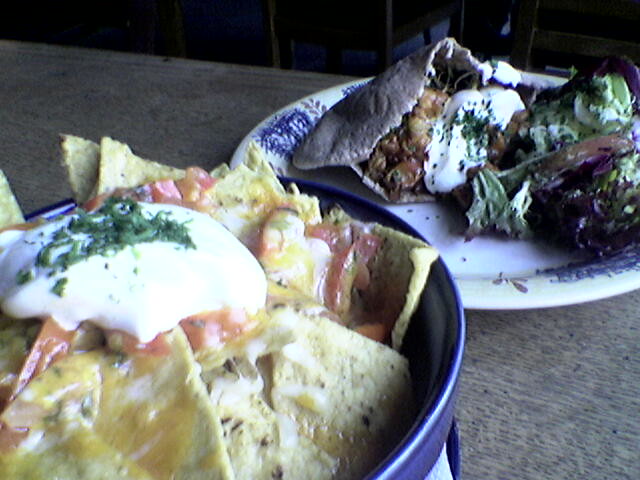The photograph captures a pre-meal scene featuring two distinct dishes set atop a wooden table, against the backdrop of a dimly lit restaurant. Prominently displayed in the foreground is a blue bowl containing yellow tortilla nachos draped in a melted Colby Jack cheese blend, with orange and yellow hues. The nachos are garnished with red tomato salsa, a generous dollop of white sour cream, and sprinkled with green herbs, either chives or cilantro. In the background, a white paper plate with blue decorative edges holds a fresh green salad of mixed greens. Adjacent to the salad is a Mediterranean-inspired pita stuffed with a yellow vegetable mix or possibly meat, also topped with sour cream or tzatziki, and finished with a sprinkle of green herbs.